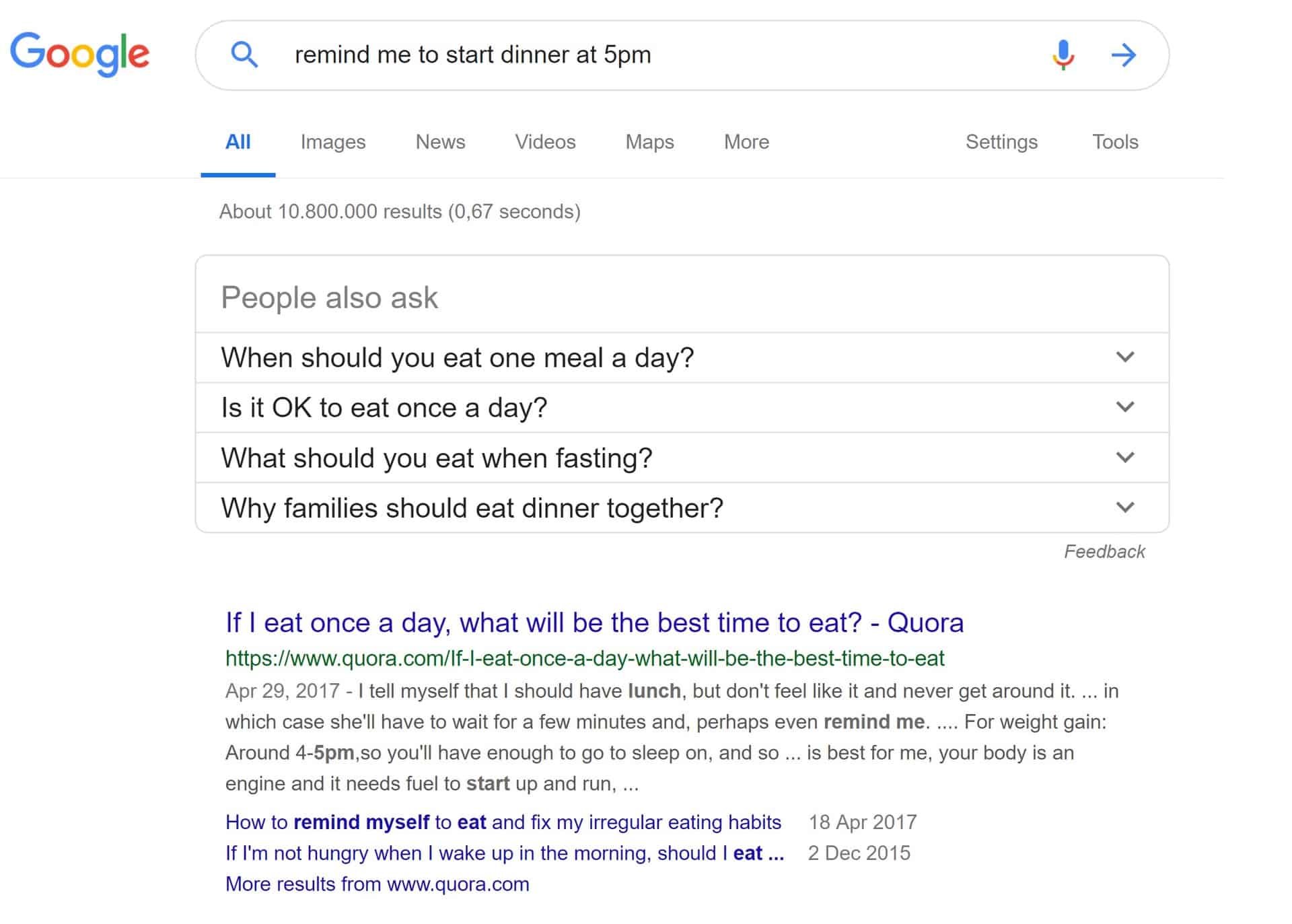In the top left corner of the image, the word "Google" is prominently displayed, with each letter in the logo taking a distinct color: the first 'G' is blue, the first 'O' is red, the second 'O' is yellow, the second 'G' is blue again, the 'L' is green, and the 'E' is red. To the right of the logo, a search bar is located, containing the text "remind me to start dinner at 5pm." On the far right end of the search bar, there's a microphone icon featuring the same color palette as the Google logo: blue, red, yellow, and green. Adjacent to the microphone icon is a blue arrow pointing to the right.

Below the search bar, several categories for search filters are listed horizontally: "All," "Images," "News," "Videos," "Maps," "More." There's a space separating these categories from the final two options: "Settings" and "Tools." 

Underneath these categories, the text indicates the search results: "About 10,800,000 results (0.67 seconds)." Below this line, a boxed section labeled "People also ask" lists related questions: 
1. "When should you eat one meal a day?"
2. "Is it okay to eat once a day?"
3. "What should you eat when fasting?"
4. "Why families should eat dinner together?"

This detailed description highlights the structure and content of the image, making it clear and comprehensive.